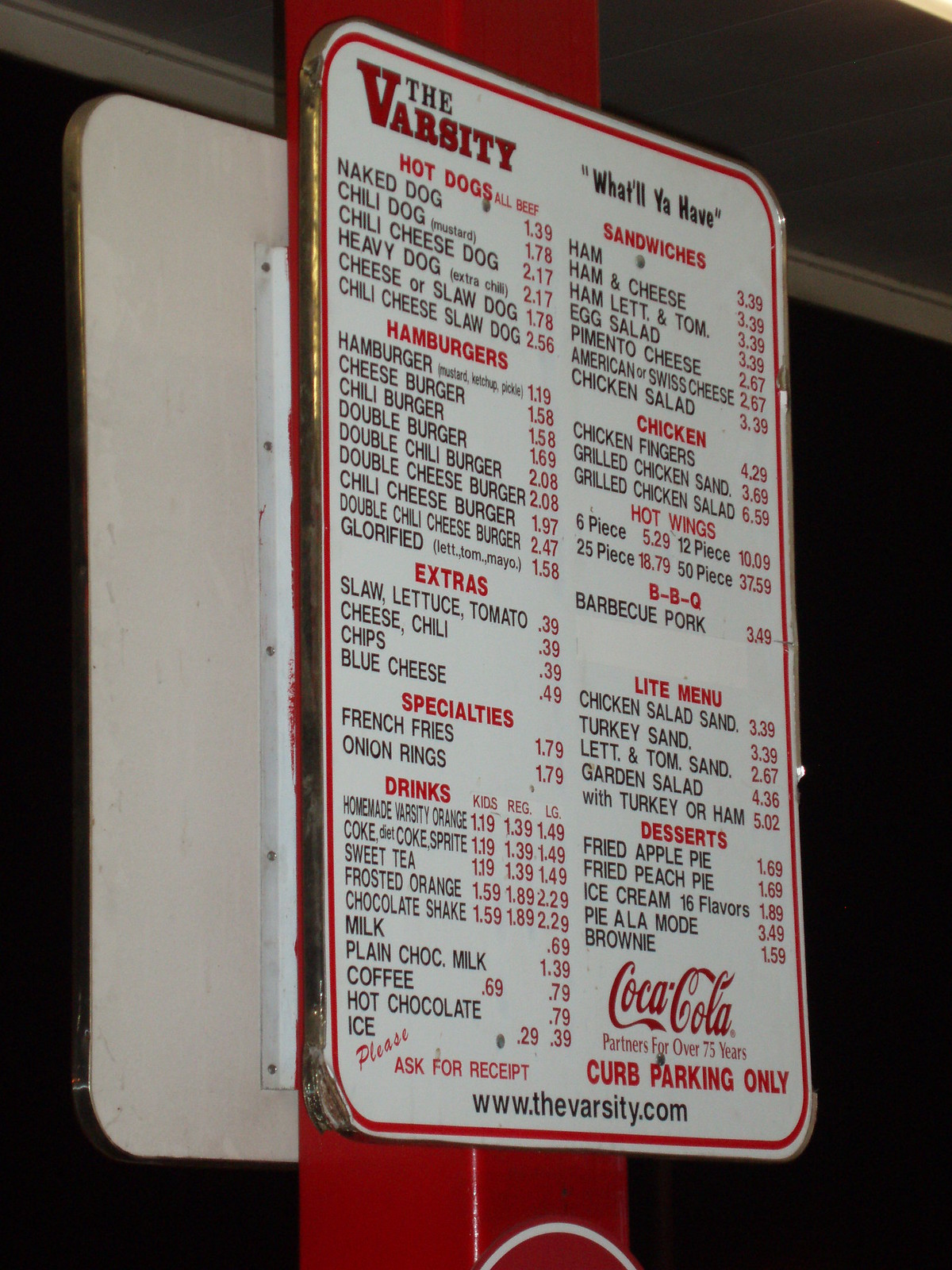The image features a prominently displayed menu from "The Varsity." The menu is presented on a metal sign mounted on a red post. The background of the sign is white with a red outline, and the text is in red and black. At the top, the sign reads "The Varsity" with the slogan "What'll ya have?" positioned to the right.

The menu is categorized into several sections. On the left column, the categories are: Hot Dogs, Hamburgers, Extras, Specialties, and Drinks. The right column includes: Sandwiches, Chicken, BBQ, Hot Wings, Light Menu, and Desserts. Each item listed under the categories has its respective price displayed in red.

At the bottom of the menu, there's a red text indicating, "Coca-Cola partners for over 75 years, curb parking only." On the left side, there's a notice that reads, "Please ask for a receipt." Finally, the web address, www.thevarsity.com, is listed at the very bottom of the sign. This detailed menu appears to be intended for a quick-service restaurant, possibly catering to sporting event attendees.